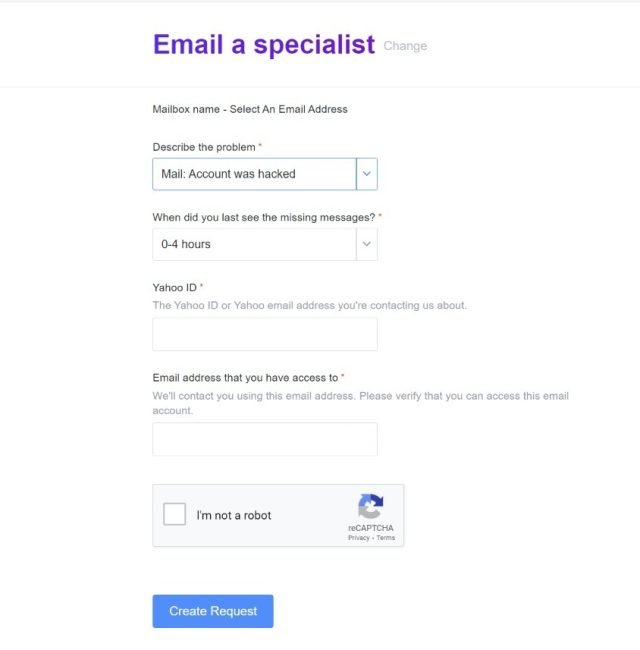The image depicts a screenshot of a form, likely on a mobile phone or computer, from a website dedicated to addressing email-related issues. At the top of the form, in purplish text, it reads "Email a Specialist," with a gray "Change" option beside it. Below this header, "Mailbox - Select an Email Address" is written in black print. 

Further down, there is a section titled "Describe the Problem" with a drop-down menu displaying the option "Mail account was hacked," which has been selected. 

Following this, another drop-down menu is present under the text "When did you last see the missing messages?" with the chosen option being "0 to 4 hours."

Vertically aligned beneath this, the form requests the user's "Yahoo ID" with the explanation "The Yahoo ID or Yahoo email address you’re contacting us about." This field is currently empty.

Subsequently, there is a field labeled "Email Address that You Have Access To," accompanied by the instruction "We’ll contact you using this email address. Please verify that you can access this email account."

Below these fields, there is a CAPTCHA checkbox labeled "I’m not a robot," followed by a button at the very bottom of the form labeled "Create Request," which users can click to submit their issue.